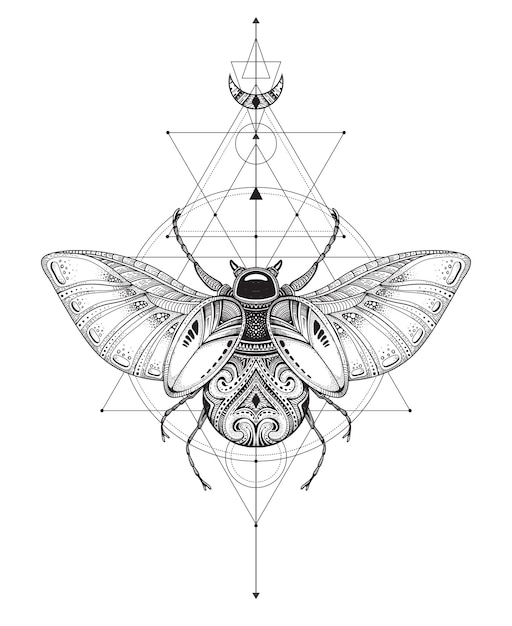This is a meticulously detailed black line drawing against a solid white background, featuring a winged insect that appears to be a beetle as the central focus. The beetle's outstretched wings extend beneath its plate-like wing covers, revealing a large abdomen adorned with intricate geometrical patterns. Its thorax is predominantly black with scattered white specks, while its shiny, helmet-like head showcases two prominent horn-like antennas. Surrounding the beetle is an elaborate pattern of fine, overlapping triangles and circles that form an intricate and ornate design. At the top of the image is a distinct crescent moon shape, adding a ritualistic and symbolic element to the artwork. The combination of multiple superimposed and inverted triangles and the clear central circle create a complex and mesmerizing background, enhancing the overall visual impact of the piece.